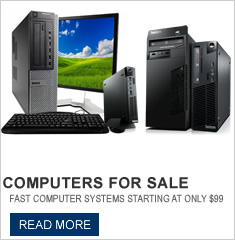In the image, there is a well-designed advertisement promoting computers for sale. The primary text of the advertisement reads, "Fast computer systems starting at only $99," which highlights the incredibly low starting price. Below this enticing offer, there is a blue box with a clickable button labeled "Read More," suggesting that more information is available for interested customers.

The visual part of the advertisement showcases four different computer towers, each varying in size, shape, and design, complete with visible CD drives. These towers are likely indicative of the diverse range of computers available for purchase, possibly varying in specifications and cost. In front of these towers, there is a standard black keyboard that includes a number pad, typical of office or home computer setups.

In the background of the setup, a monitor is displaying the classic Windows desktop wallpaper, featuring a green field under a clear blue sky. This familiar wallpaper adds to the recognizable setting of a computer advertisement. The clean layout and straightforward presentation make it clear that the focus is on the affordable and fast computer systems being promoted.